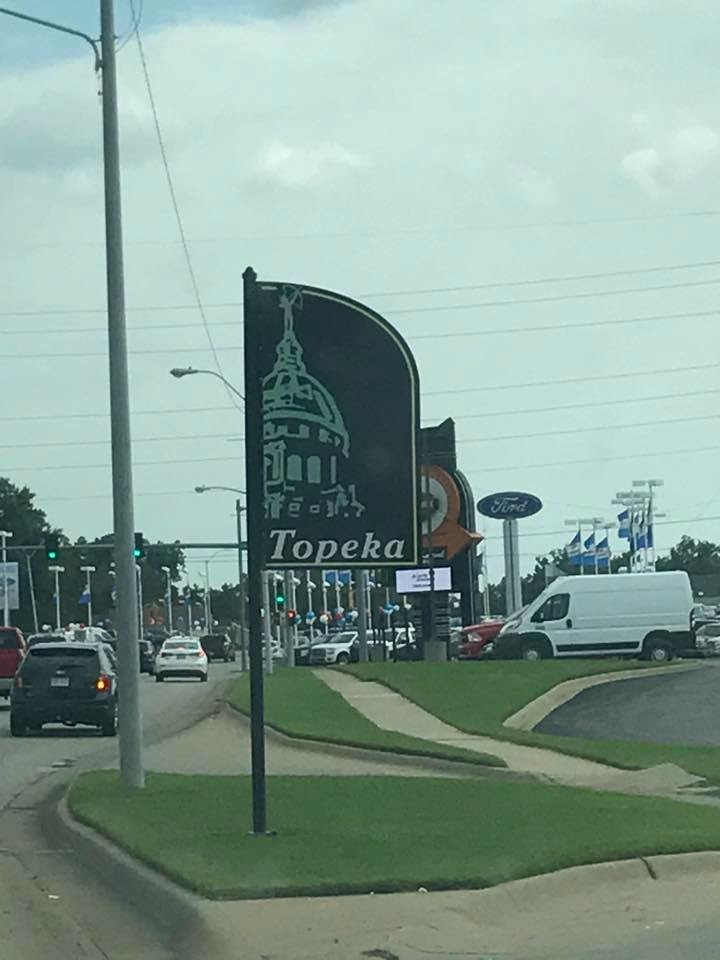This image captures a bustling street scene in Topeka, Kansas. Prominently featured is a city banner displaying an image of the Kansas State Capitol with the word "Topeka" underneath. The banner adds a charming touch to the street and hints at the city's pride in its historical architecture. To the left, several cars drive along a four-lane road, with a traffic light glowing green farther down the street, indicating the ongoing motion of city life. On the right side, a Ford dealership is visible, distinguished by a large Ford sign, colorful balloons, and rows of neatly arranged cars in the parking lot. The sky is overcast with thick, gray clouds, giving the scene a gloomy, almost rainy atmosphere. The state capitol depicted on the Topeka banner has a sage-green hue set against a darker, almost black, background, evoking a sense of vintage charm.